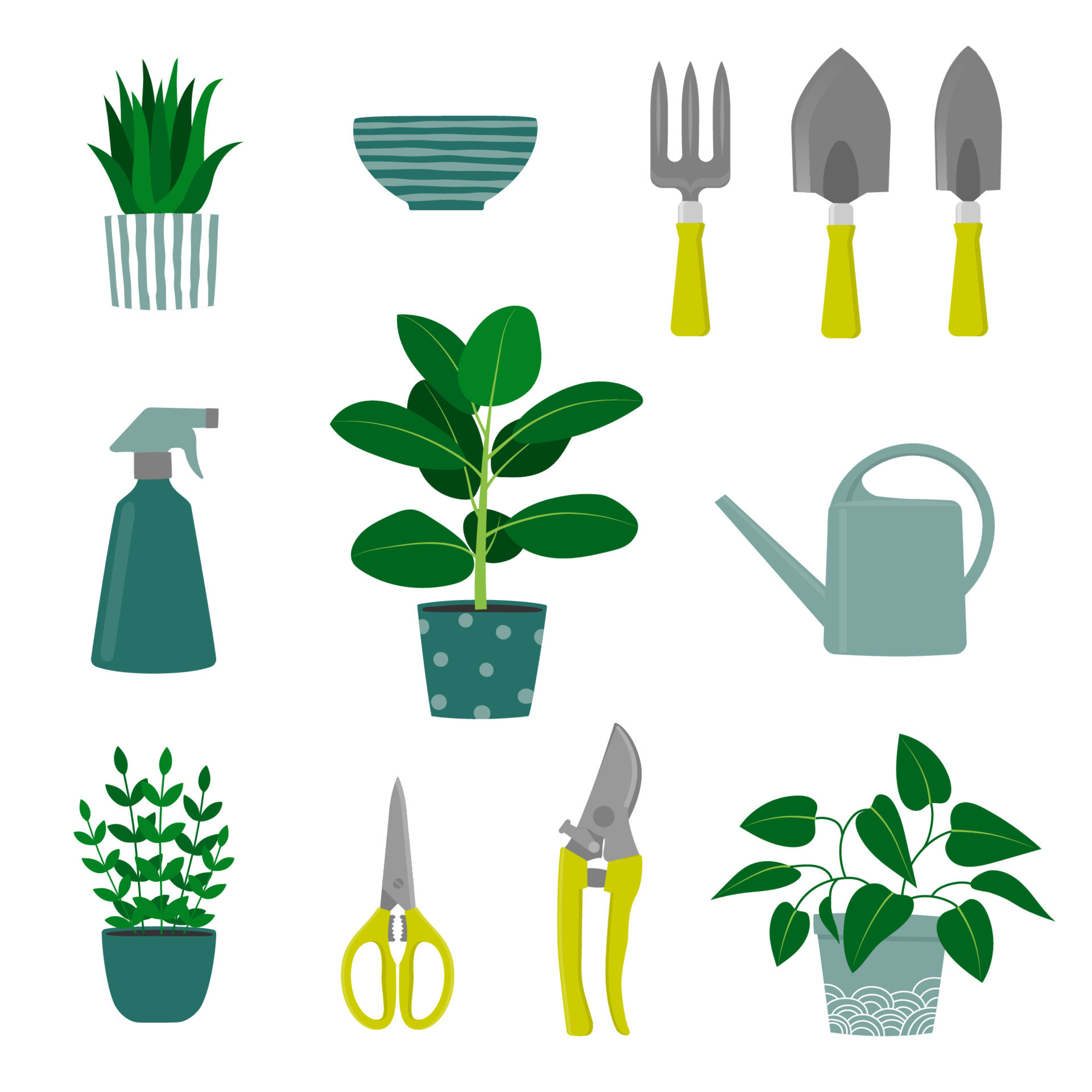The vertical rectangular image depicts a detailed and artistic arrangement of gardening tools and potted plants in organized rows of three. On the top left, an aloe vera plant in a pot with white and green vertical stripes is prominently featured. Adjacent to it is a light green spray bottle with a gray opening. Other tools in this row include items typical for gardening, all with yellow handles.

In the middle row, the central focus is a green pot with gray polka dots, housing a growing plant. It is flanked by a green spritz bottle and a watering can, reflecting the practical tools used for plant care. In the bottom row, a green plant is situated to the left, followed by a pair of scissors with yellow handles and a cutter with matching yellow handles, ending with another potted plant.

The entire scene gives an impression of garden emojis or a digital NFT creation with its bright colors and delicate handiwork, potentially aimed at teaching or engaging children in gardening. Each tool and plant, carefully rendered, collectively creates a visually appealing and organized display.